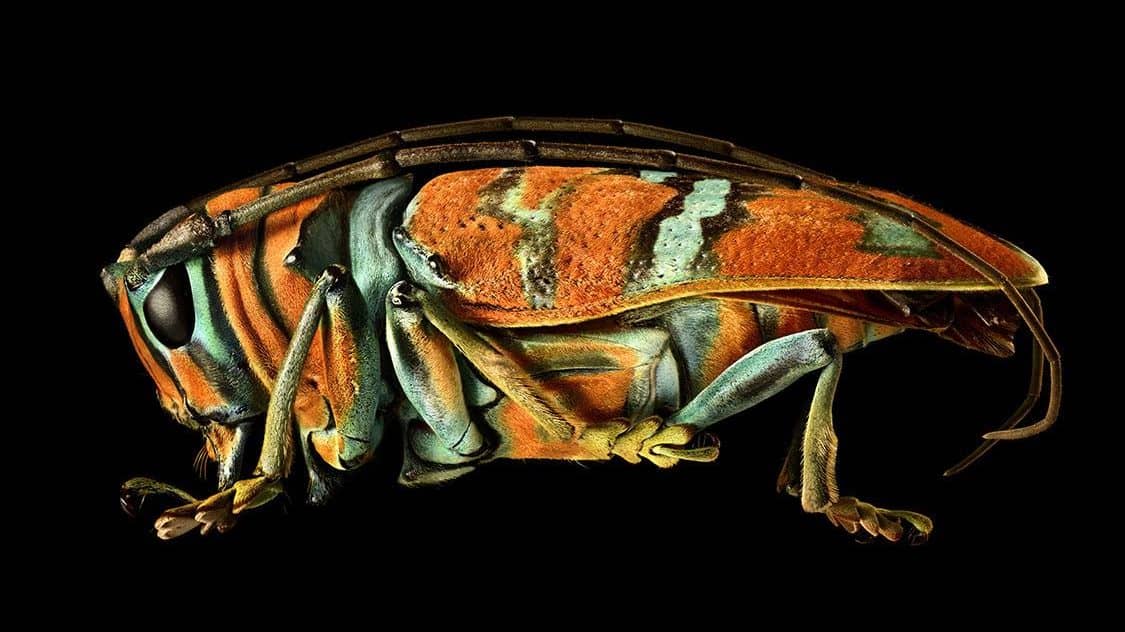The image is a close-up of an insect resembling a grasshopper or a cricket, showcased against a black background. The insect is captured in a left-side profile, exhibiting a body that is somewhat short and squatty in length. It features a striking tiger-like pattern with orange, white, and black stripes running vertically across its entire body. The large, black eyes are prominent, with subtle black and white striping around them. From just above the eyes, two long antennae extend backward along the length of the body and curl slightly at the end. The insect’s legs are crinkled and positioned as if poised to hop, with intricate layers of skin visible on its feet. Tiny hairs sprout around its small mouth, adding to its detailed appearance. The segmented body displays a clear distinction between the head and the rest of the torso, and despite the unusual coloration and proportions, the overall look of the insect appears exotic and almost unreal.